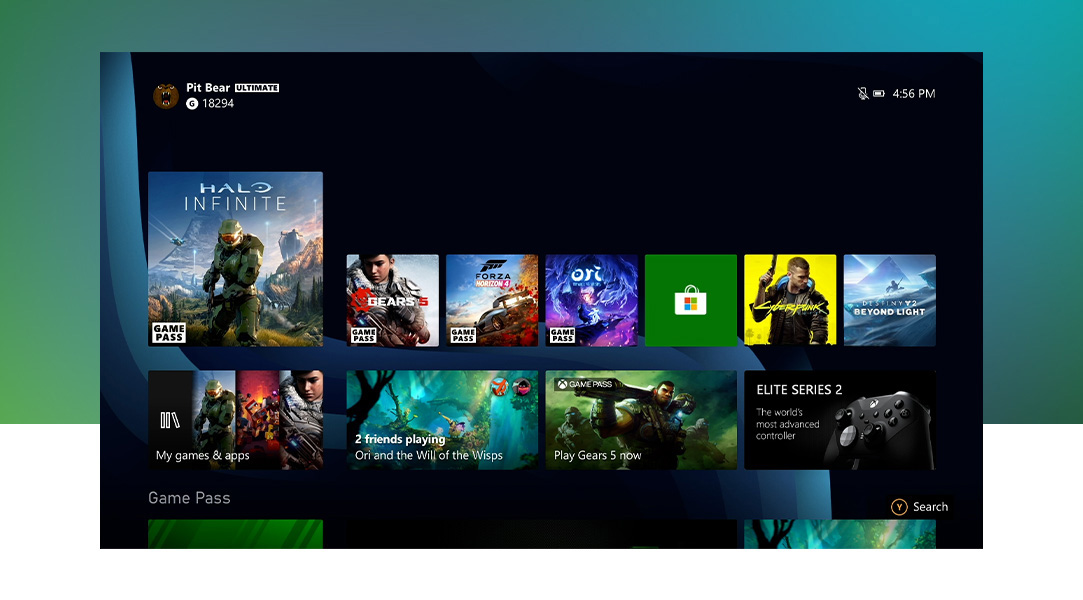The screenshot taken from a device screen showcases a multi-layered interface filled with vibrant imagery and detailed text. The backdrop features a horizontal rectangular gradient transitioning from various shades of blue on the right side to greens and almost yellow hues on the bottom left.

In the forefront, a prominent black rectangle occupies the center of the screen. In the top area of this black rectangle, the user name "PitBear" is displayed. Below the user name, a white rectangle reads "Ultimate," and beneath it is the number "18294." On the right side of the screen, indicators in white show that the microphone is off, the battery level, and the current time, 4:56 PM.

At the bottom of the central black rectangle, white text spells out "Game Pass." Directly below this, a green rectangle is present. In the bottom right-hand corner, there's a pull-down menu labeled "Search." Beneath this is a mottled blue and green rectangle featuring a black, tree-like object.

On the left-hand side of the screen, two sweeping blue lines run diagonally through the background. The middle of the screen is populated by rows of various video game images. The first four images in the top row have "Game Pass" indicated in the bottom left corners. These include "Halo Infinite," "Gears 5," "Forza," and "Ori (O-R-I)."

Adjacent to these game images, a green rectangle with a Google Shopping bag icon appears, followed by an image for "Cyberpunk," and on the far right, an image for "Destiny Beyond Light."

In the row beneath, there is an image labeled "My Games and Apps," with text indicating "Two Friends Playing Ori and Will of the Wisps." Next to it, another section with "Game Pass" promotes playing "Gears 5." On the far right of this row, there's an advertisement for the "Elite Series 2," described as "the world's most advanced controller," illustrated with a picture of a sleek black controller.